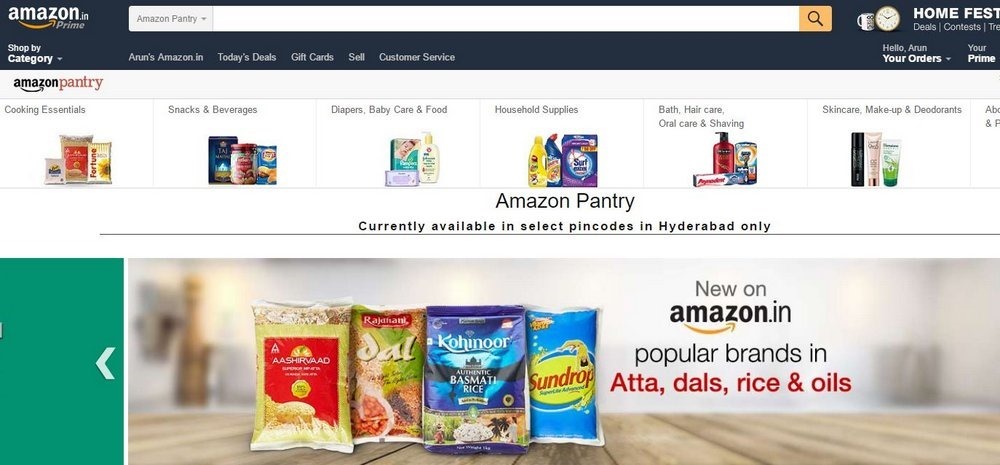This is a screenshot from the Amazon Pantry webpage, specifically tailored for users in Hyderabad. The page features a variety of categories including cooking essentials, snacks and beverages, diapers and baby care products, food items, household supplies, and personal care products such as bath, hair, oral care, shaving, skincare, makeup, and deodorants. A prominent section highlights that Amazon Pantry services are currently limited to select pin codes in Hyderabad only. Additionally, the page promotes new arrivals on Amazon.in and showcases popular brands in categories such as Atta, Dals, Rice, and Rolls. 

At the top of the page, the Amazon navigation bar includes the logo followed by options such as Prime, Shop by Category (with a dropdown menu), Amazon.in, Today’s Deals, Gift Cards, Sell, Customer Service, Home Fest, and a personalized greeting with the user’s name, Arun, directing to 'Your Orders'. The page is visually engaging with a palette consisting of blue, yellow, red, white, black, tan, green, brown, orange, purple, mauve, gold, and pink.